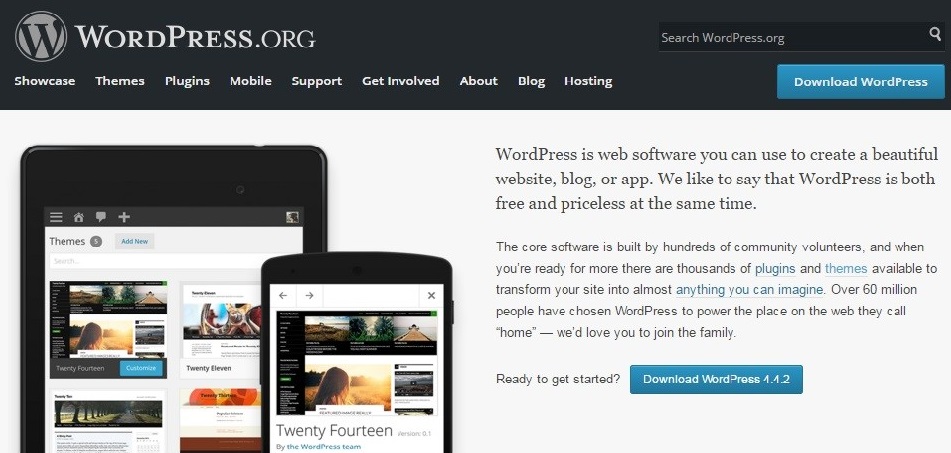Screenshot of the WordPress.org homepage featuring a sleek, user-friendly design. The top section displays a black navigation bar containing links for Showcase, Themes, Plugins, Mobile, Support, Get Involved, About, Blog, and Hosting. In the top right corner, a search bar is visible. Below the navigation bar, a large blue button labeled "Download WordPress" stands out prominently.

The main content area centers on an illustrative image showcasing both a tablet and a phone, each displaying a sample website to highlight the platform's ability to seamlessly create both desktop and mobile versions of a site. Accompanying this visual is a compelling tagline: "WordPress is web software you can use to create a beautiful website, blog, or app. We like to say that WordPress is both free and priceless at the same time."

Further text elaborates on the platform's robust foundation, noting that its core software is developed by hundreds of community volunteers. Additionally, users can enhance their websites with thousands of available plugins and themes. For users ready to jump in, another blue button encouraging them to "Download WordPress 4.4.2" is prominently featured. This platform serves as either a customizable framework for developers or an all-in-one service for those looking to have their website ready to go, offering extensive options for personalization in terms of both aesthetics and functionality.